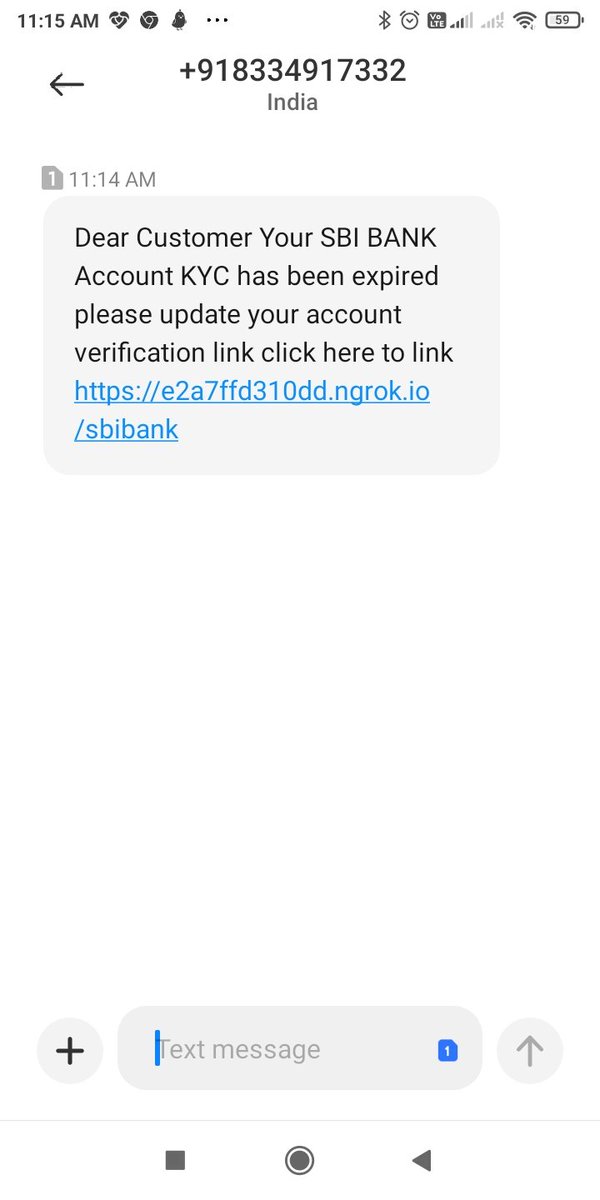The image depicts a screenshot of a message on a cell phone. At the top of the screenshot, the status bar displays the time "11:15 AM," along with several icons and three dots indicating additional settings or notifications. The battery life is also shown. Below the status bar, there is a back arrow pointing to the left, followed by a phone number from India, formatted as "918-334-917-332." The body of the screenshot captures a message received at "11:14 AM," within a speech bubble that reads: "Dear customer, your SBI bank account KYC has expired. Please update your account verification link, click here to link." Following this text is a clickable HTTPS link, highlighted in teal and underlined.

There is a considerable amount of blank space following the message. At the bottom of the screen, there's an input area where a reply text message can be sent, characterized by a blue line indicating where the user could start typing. The very bottom of the image features three touch-sensitive navigation icons: a square, a circle, and a triangle.